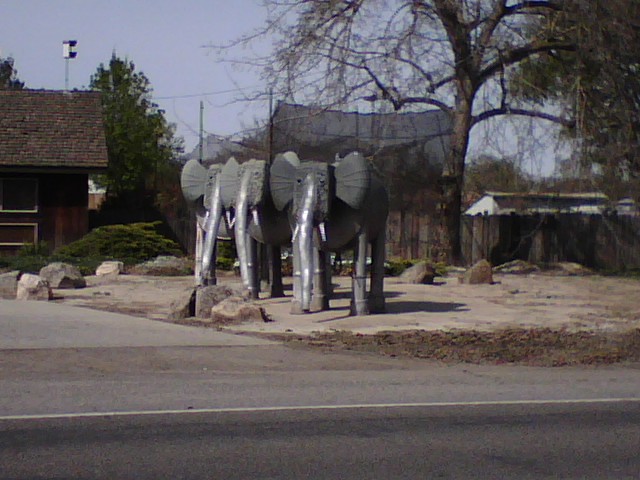The photo captures a distant view of three distinctive metallic elephant sculptures, positioned on the opposite side of a two-lane street. Each sculpture features trunks hanging down to the ground, crafted from shiny, silver metal tubes resembling pipes. The legs of the elephants are constructed from multiple chimney-like tubes, while their bodies appear to be made from large, metal barrels. The ears protrude noticeably and the faces, with holes for eyes, are fashioned from a darker metal. Each elephant boasts two metal tusks.

In the background to the left, there's a small, weathered brown house with an angled roof covered in shingles. The house has an antenna-like structure on top, and in front, there is a gravel driveway scattered with boulders. Behind the elephants, a large tree with sparse branches can be seen, and to the right of the photo is a trampoline encircled by netting. The scene also includes an old, brown wooden fence that stretches across the right side, with another building visible in the distance which hosts a birdhouse-like structure on its roof. The entire setting is outdoors, bathed in natural light, under a blue sky, giving a clear view of the unique and whimsical sculptures along with their surroundings.